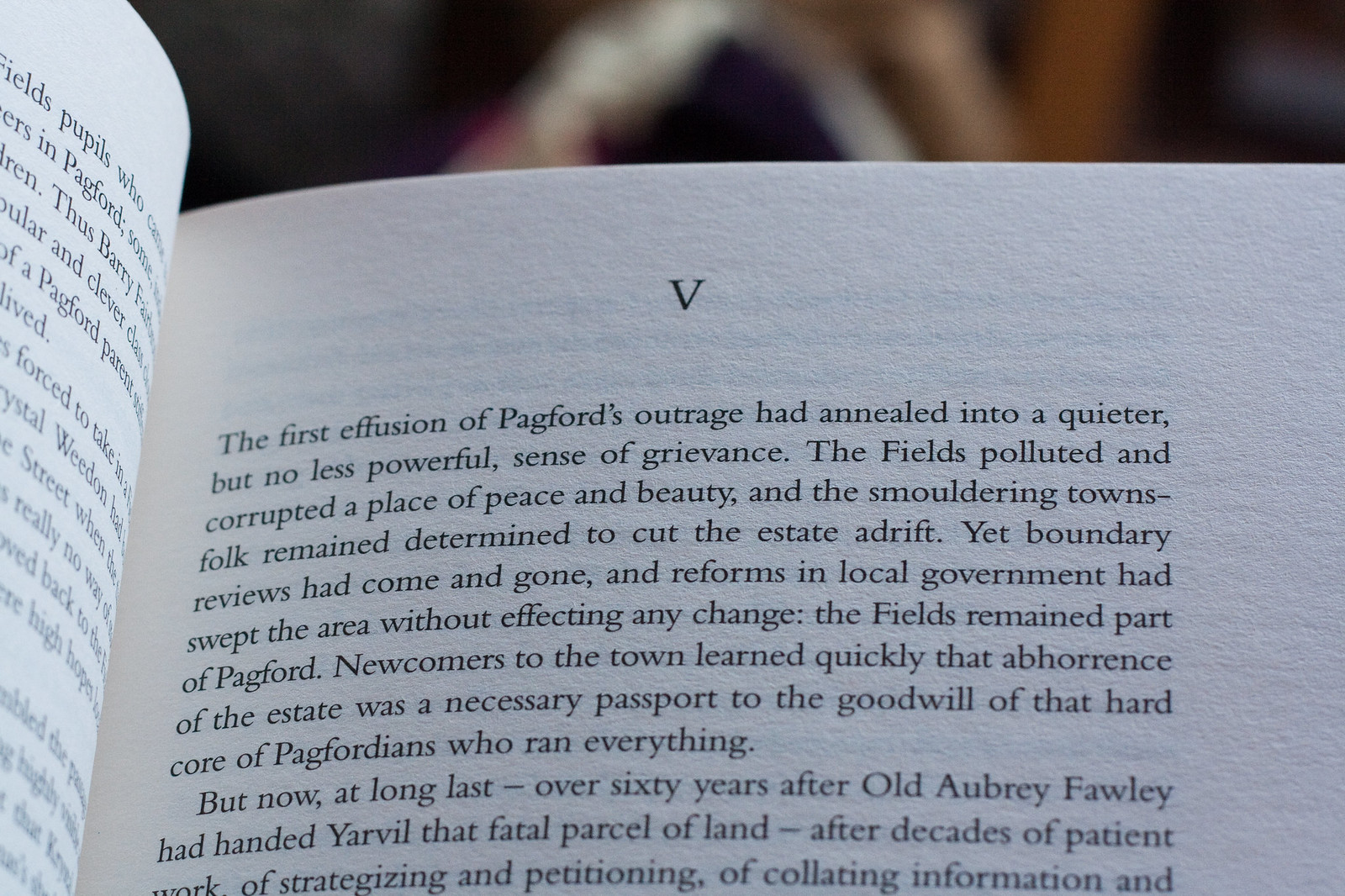This image focuses on the upper portion of the right page of an open book, specifically the top third. The page is crisp and clean, indicating the book is relatively new. The content starts with the Roman numeral "V," suggesting it is from the fifth chapter. The legible text reads: “The first effusion of Pagford's outrage had annealed into a quieter, but no less powerful, sense of grievance. The fields polluted and corrupted a place of peace and beauty, and the smoldering townsfolk remained determined to cut the estate adrift. Yet boundary reviews had come and gone, and reforms in local government had swept the area without effecting any change. The fields remained part of Pagford. Newcomers to the town learned quickly that abhorrence of the estate was a necessary passport to the goodwill of that hardcore of Pagfordians who ran everything. But now, at long last, over 60 years after old Aubrey Fawley had handed Yarville that fatal parcel of land, after decades of patient work of strategizing and petitioning, of collating information and…”

The surrounding background is heavily out of focus, making it indiscernible, which accentuates the book as the primary subject. The font is a classic black serif on a pristine white page, further enhancing the book's fresh appearance. Given the narrative style and content, the passage likely comes from a novel.